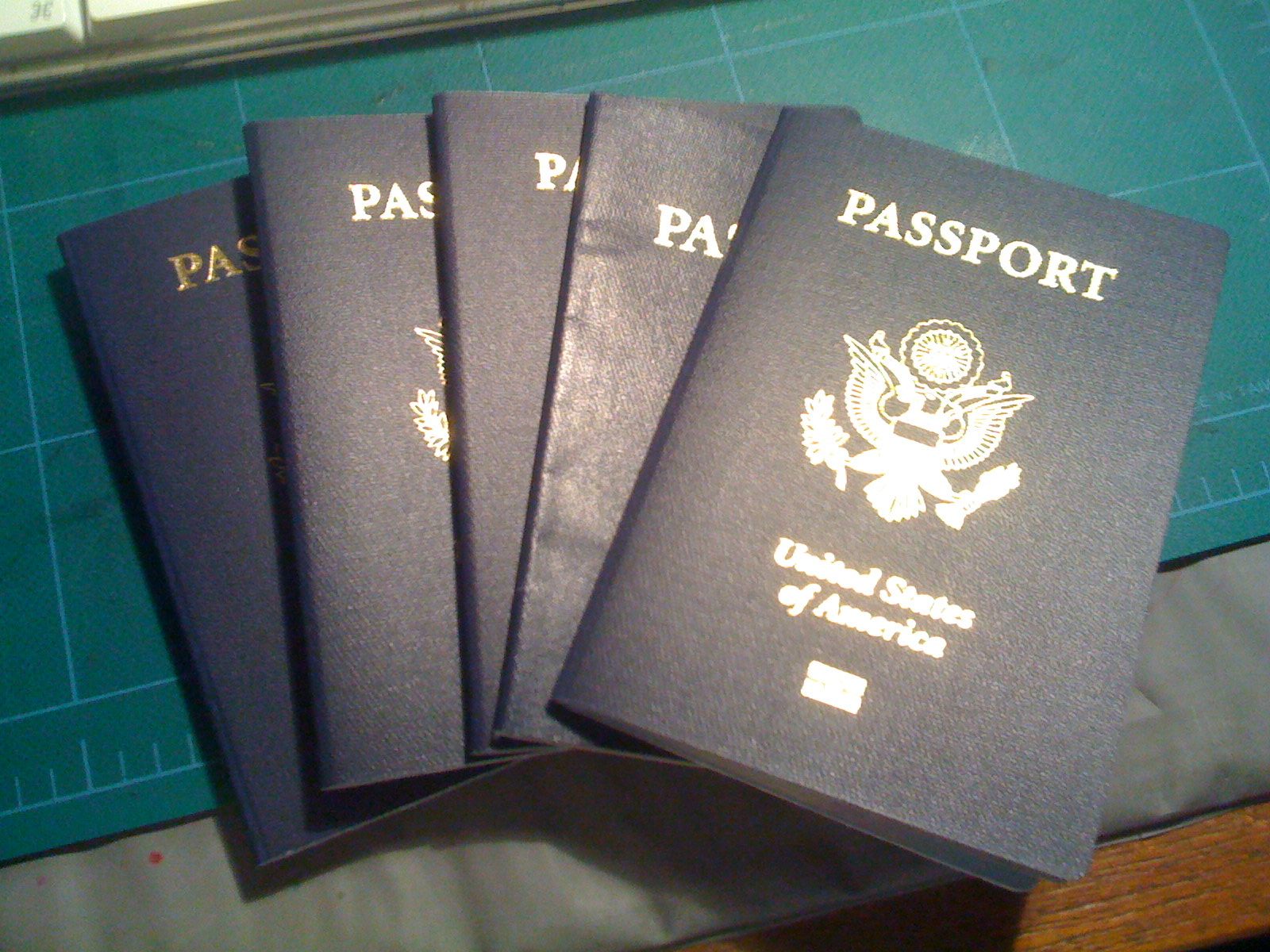In this detailed photo, we observe a stack of five U.S. passports arranged in a staggered manner, reminiscent of a spread deck of cards. The passports are placed on each other in such a way that only a sliver of each cover remains visible. The passport at the top of the stack features a dark blue cover with gold lettering, reading "passport" at the top, an eagle emblem in the center, and "United States of America" below it, all reflective of an overhead light. The next three passports, judging by their visible upper edges, appear to be a lighter shade of blue with similar designs, but the lettering is rendered in silver. The fifth passport, peeking out at the bottom, maintains the same reflective quality, albeit with a more subdued shade perhaps due to lighting.

This entire stack is resting on top of a green piece of fabric that displays a grid pattern, suggesting an architectural or design-oriented surface. Below this green fabric, there's another piece of fabric with a grayish hue, potentially a bed sheet or something similar, adding another layer of texture. All of these layers—passports and fabrics—are situated on a wooden table, the grain of which is faintly visible around the edges of the stack.